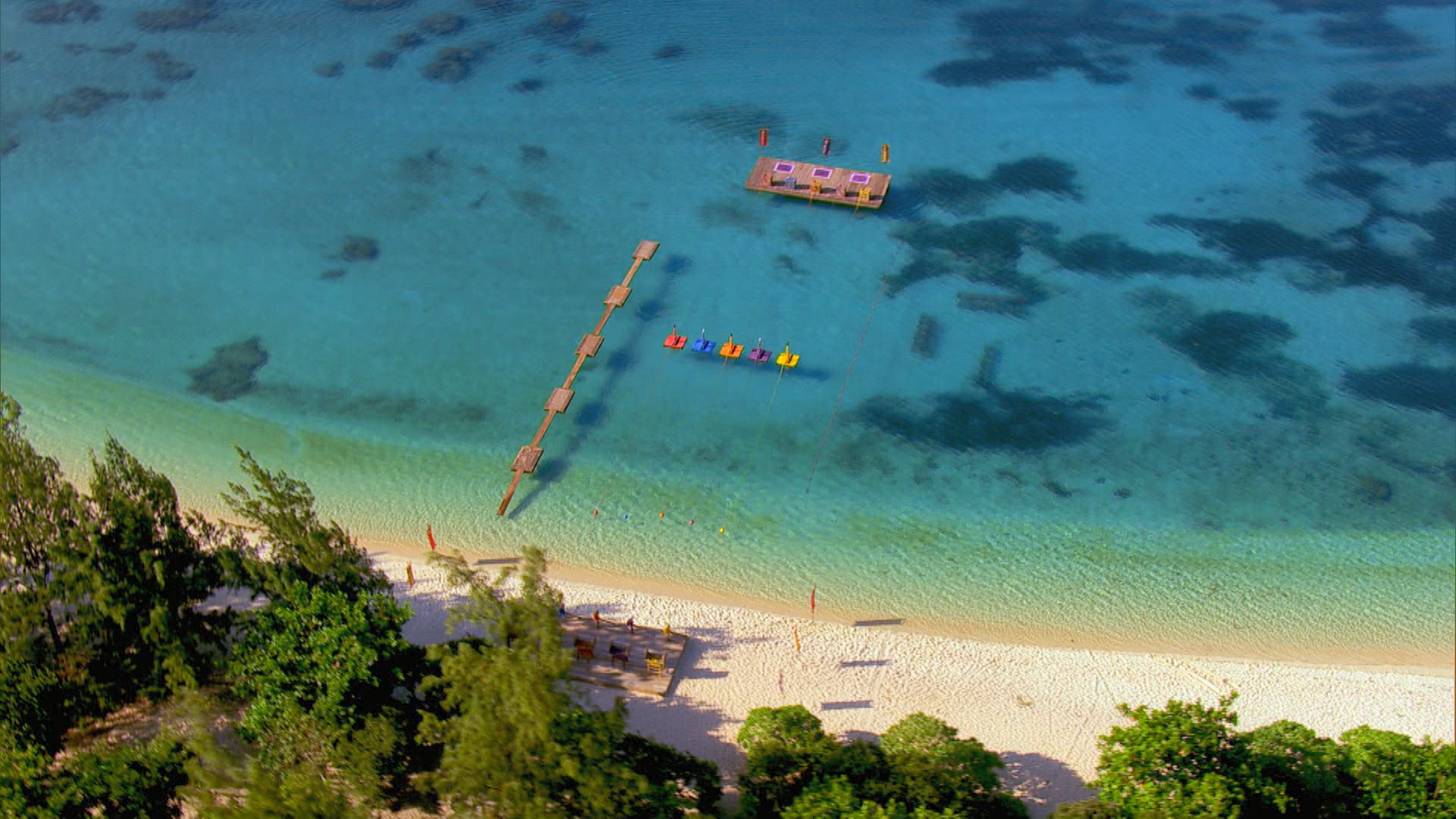This aerial drone shot captures a picturesque tropical beach scene with stunning, clear blue water. At the bottom of the image, lush green trees line the sandy shore, transitioning into a pristine beach. Extending from the beach, a narrow floating pier stretches out into the sea, accompanied by a series of neatly arranged, brightly colored platforms in red, blue, orange, purple, and yellow. These small platforms may serve as seating or sunbathing spots. The water's exceptional clarity reveals darkened areas beneath the surface, possibly indicating rocky formations or coral reefs. Out further into the water, a larger floating platform suggests preparations for a potential athletic event, like swimming races, although no participants are visible in the shot. The beach also features some kind of setup with tables and banners, adding to the event-like atmosphere.